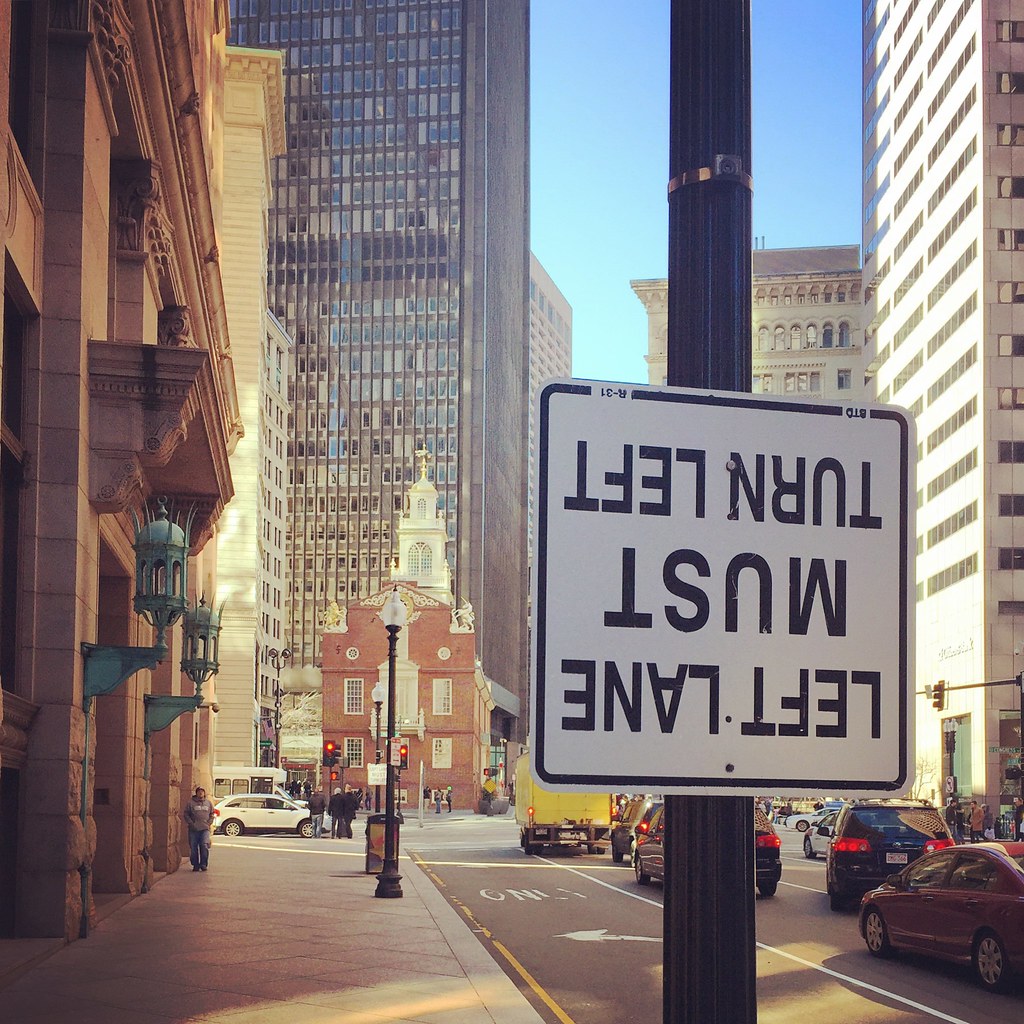The image depicts a bustling city street, possibly in New York, featuring a central black street pole with an upside-down white traffic sign bordered in black. The sign, written in black text, reads "Left Lane Must Turn Left." Surrounding this, to the left, is a brown building adorned with large, blue-gray street lamps, while farther left and to the bottom right are several cars on the road. A large sidewalk extends along the left side of the image, with the road itself marked with "Only Left Turn" in white text. In the background, towering skyscrapers with numerous shiny windows reach into a clear, blue sky, and one notable building features large arched windows. Sunlight streams in, brightly illuminating the tall building on the right.